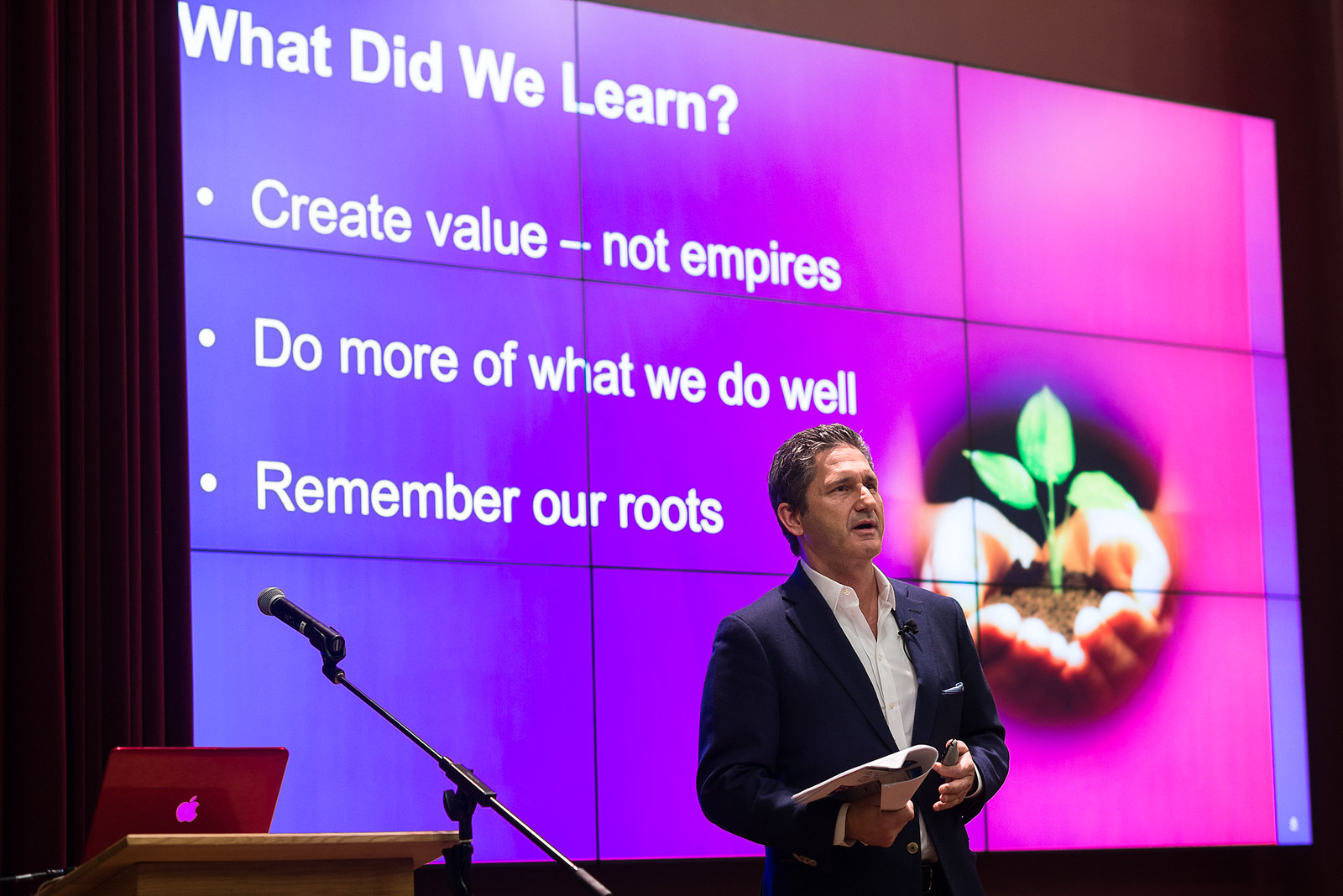In the image, a distinguished older man, likely in his late 50s, is giving a presentation. He is speaking to an audience off-camera, dressed in a dark blue suit paired with a white button-down dress shirt. A microphone is attached to his suit, and he holds a piece of paper in his right hand. His short brownish-gray hair and confident demeanor suggest he is an executive. 

Behind him is a large projector screen featuring a vibrant background that transitions from purple on the left to pink on the right. At the top left of the screen, white text reads, "What Did We Learn?" Beneath the title are three bullet points: "Create Value - Not Empires," "Do More of What We Do Well," and "Remember Our Roots." On the right side of the screen, there is an image of hands cupping a pile of dirt with a green sapling emerging, which has three leaves.

To the left of the man, there is an empty wooden podium with a red-cased MacBook on it, and a microphone stand positioned nearby. A red curtain frames the left side of the image, completing the scene of a formal and instructive presentation.